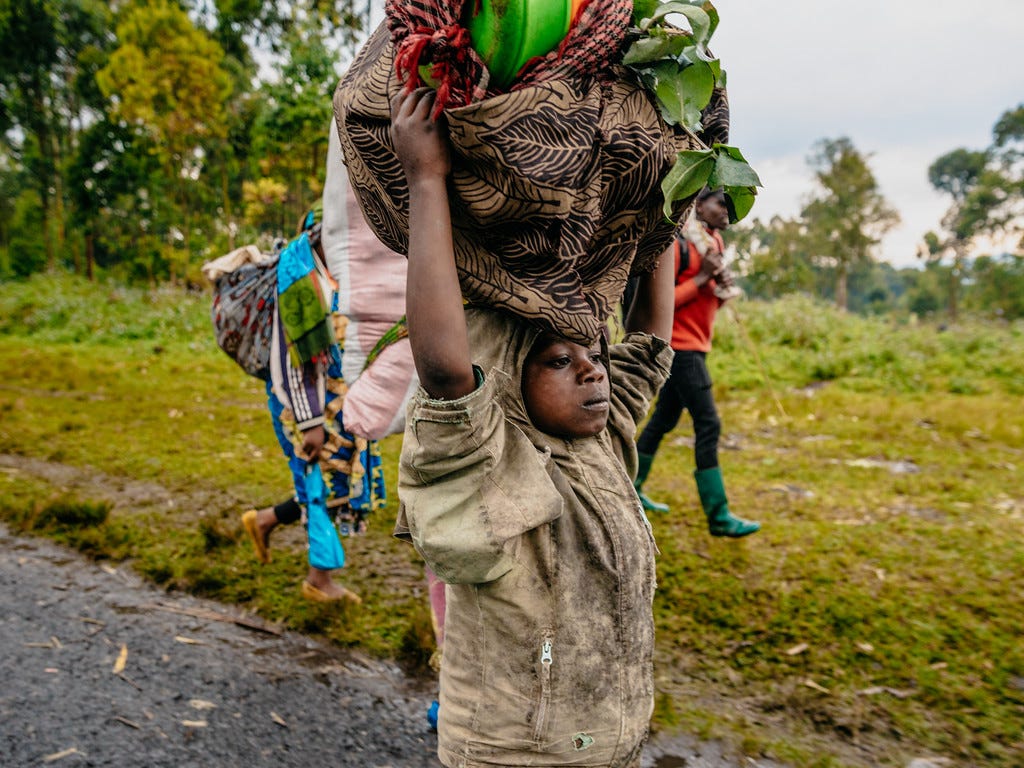In this outdoor photograph, a young boy, likely African and appearing impoverished, is walking from left to right on what looks like a wet dirt road. He is dressed in a worn, ripped, and dirty beige-brown coat and balances a large bundle on his head, wrapped in a cloth. From the bundle, green leaves protrude, suggesting it contains some kind of plant or food. The scene is set under a gray, cloudy sky, which complements the wet ground, hinting at recent rain.

To his right and slightly ahead, another person walks on a grassy area, donning an orange jacket, black pants, and black boots. Just behind him on the left, another figure, possibly carrying a similar bundle, follows. In the background, a blur of green trees and grass, indicative of a forest-like area, frames the scene, further enhancing the rural and impoverished setting. All elements focus on the boy at the center, emphasizing the hardship and resilience in his expression and posture as he navigates this rural landscape.